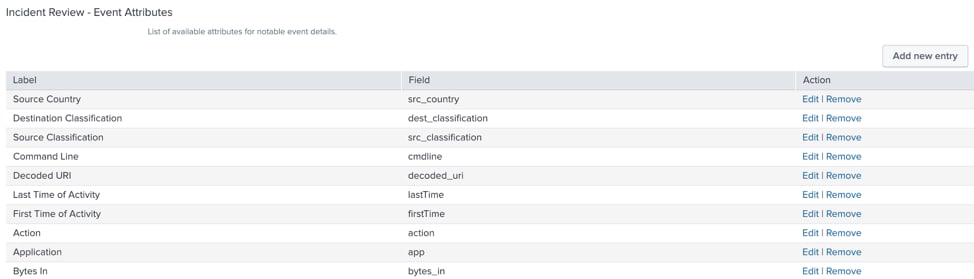Here is a detailed and cleaned-up caption based on the provided voice description:

---

The image is a clear and readable screen capture of an interface, titled "Incident Review Event Attributes" displayed at the top in black font. Below the title, there is a section labeled "List of Available Attributes for Notable Event Details" that organizes information into columns. 

The interface contains several rows, where each row includes labels and corresponding fields, colored in gray, followed by action options "Edit" and "Remove" in blue. At the top of this list, a box labeled "Add New Entry" is visible.

The following attributes and their respective fields are listed sequentially:

- Source Country: `SRC_country`
- Desensitization Classification: `DST_classification`
- Source Classification: `SRC_classification`
- Command Line: `CMD_line`
- Decoded URL: `decoded_URL`
- Last Time of Activity: `last_time`
- First Time of Activity: `first_time`
- Action: `action`
- Application: `app`
- Bytes In: `bytes_in`

Each of these rows has "Edit" and "Remove" options next to them. The font in the image is small but clear and legible. There are no additional images, pixelation, or blurring in the screenshot.